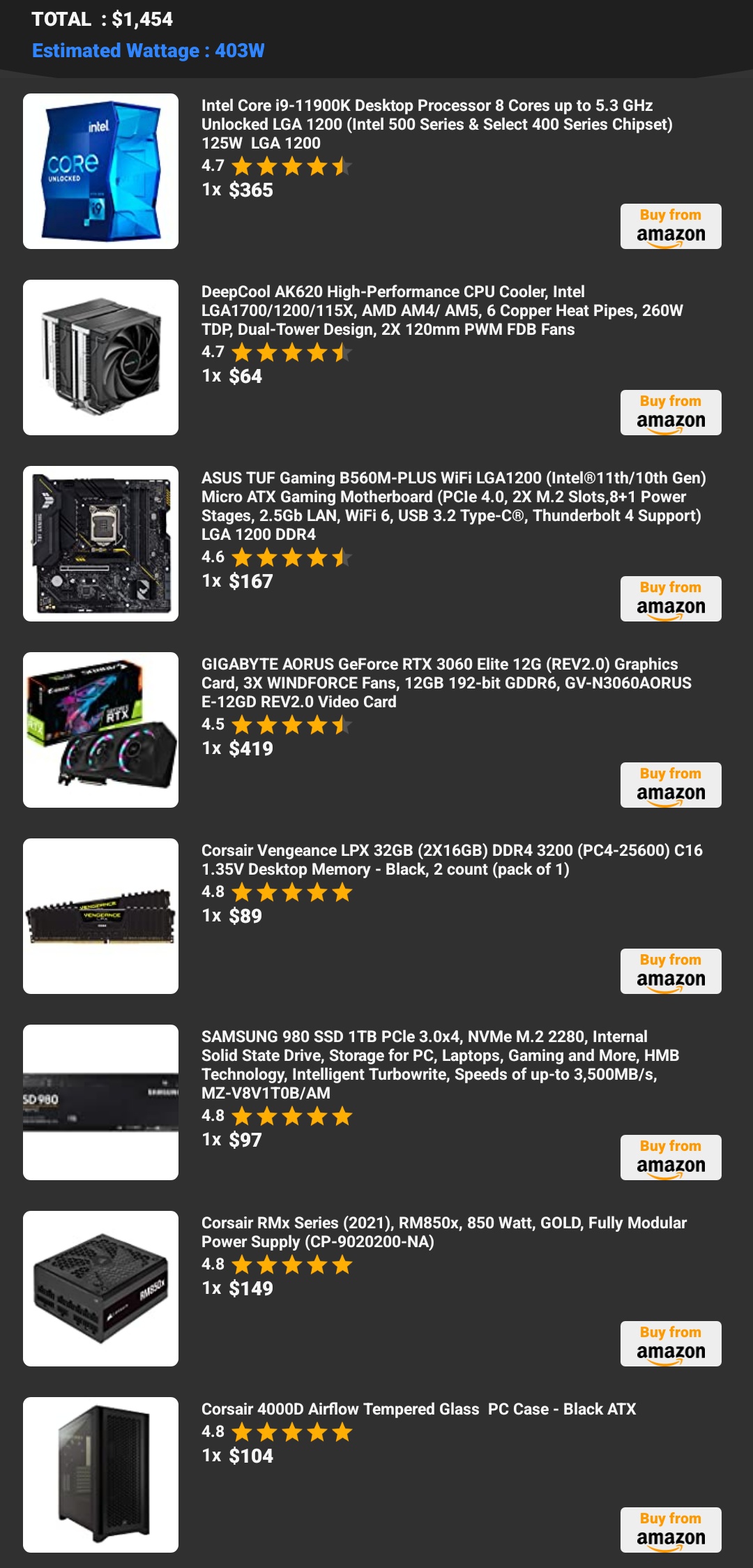This image depicts a vertically oriented screen, likely from a cell phone, displaying a list of eight items available for purchase on Amazon, set against a black background. At the top left corner of the screen, in white text, the total cost is indicated as $1,454. Just below, in blue text, the estimated wattage is listed as 430 watts.

The items are displayed in a list format with each one comprising a color photograph on the left side, framed by a white square, and a detailed description to the right. Below each description, on the bottom right, there is a white “Buy from Amazon” button. Here's a comprehensive breakdown of the items from top to bottom:

1. **Intel Core i9 11900K Desktop Processor**: Featuring 8 cores and speeds of up to 5.3 GHz, this item has a rating of 4.7 stars, with 1 unit available for $365.
   
2. **DeepCool AK620 High Performance CPU Cooler**: This cooler, rated 4.7 stars, is available for $64.

3. **Asus TUF Gaming B560M Plus Wi-Fi LGA 1200 Intel 11th/10th Gen Micro ATX Gaming Motherboard**: This motherboard has a 4.6-star rating and is priced at $167.

4. **Gigabyte AORUS GeForce RTX 3060 Elite 12GB Graphics Card**: With a rating of 4.5 stars, this graphics card is listed for $419.

5. **Corsair Vengeance LPX 32GB RAM**: Rated 4.8 stars, this RAM is available for $89.

6. **Samsung 980 SSD, 1TB**: This solid-state drive holds a 4.8-star rating and costs $97.

7. **Corsair RMX Series Power Supply**: This power supply unit is rated 4.8 stars and is listed for $149.

8. **Corsair 4000D Airflow Tempered Glass PC Case**: With a 4.8-star rating, this PC case is available for $104.